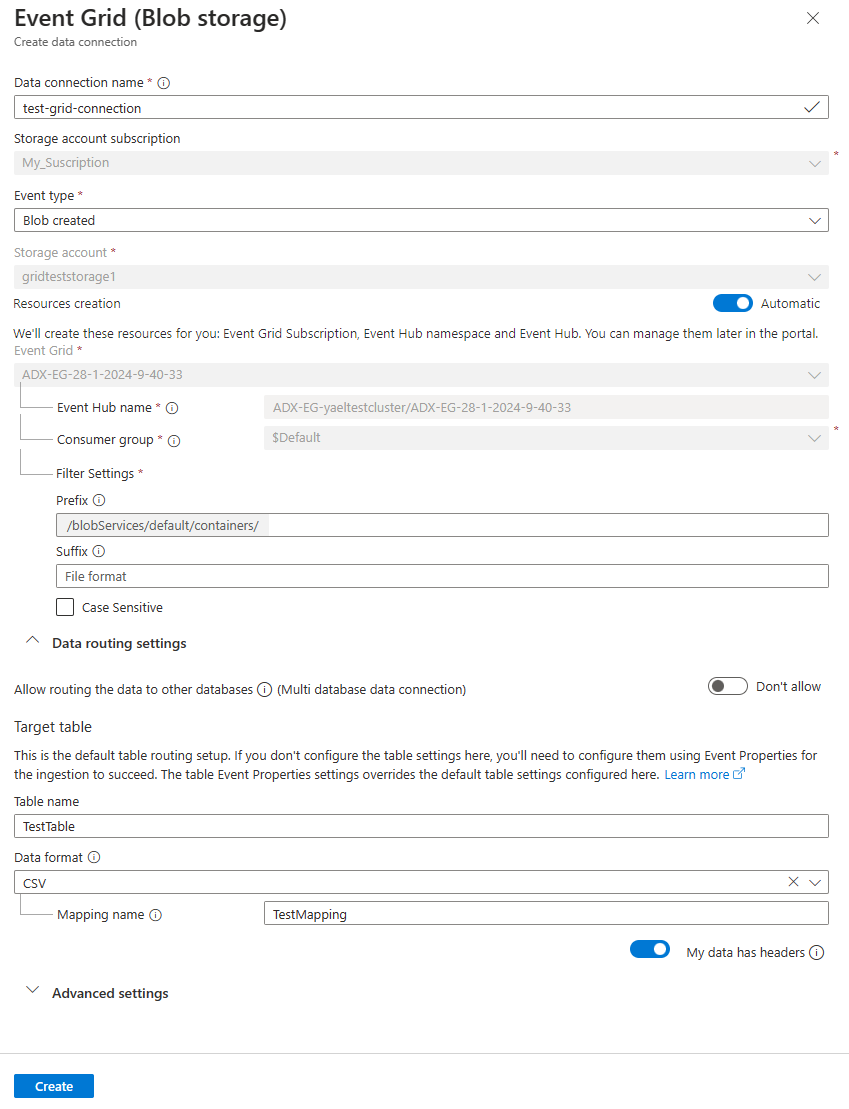In this image, we see a detailed interface of a web page that appears to be from a settings or configuration dashboard, primarily white with light gray accents. 

### Top Section:
- **Top Left Corner**: Displays the heading "Event Grid (Blob Storage)".
- **Main Control Panel**: Features an option to "Create Data Connection".
    - **Data Connection Name**: An input bar for users to enter the name of the data connection.
    - **Storage Account Subscription**: Another input bar for subscription details.
    - **Event Type**: A drop-down menu for selecting the type of event.
    - **Storage Account**: An associated drop-down menu for storage account selection.

### Mid Section:
- **Resource Creation Section**: Instructions and options for resource creation, including:
    - "Recreate These Resources For You: Event Grid, Event Hub, Namespace, and Event Hub".
    - Options can be toggled on and off, and input fields are available for:
        - Event Hub Name
        - Consumer Group
        - Filter Settings with Prefix, Suffix, and other case-sensitive parameters.

### Bottom Section:
- **Routing and Table Configuration**:
    - **Allow Routing to Other Databases**: A toggle option for Multi-Database Connection.
    - **Target Table Description**: An explanation that this section concerns the default table routing setup:
        - If not configured here, properties must be set via Event Properties for successful data ingestion.
        - Overrides feature for table and property settings, with a "Learn more" link.
        - Options for Table Name, Data Format, Test Map.

### Very Bottom:
- **Advanced Settings**: A link to advanced settings and a note regarding free access.

The layout is structured to guide users through setting up data connections and configuring necessary settings for event handling and storage management.